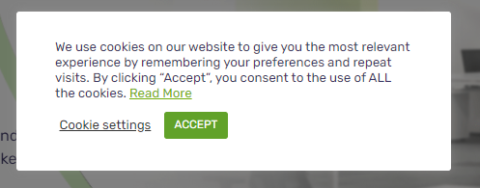In the image, the focus is on a large rectangular notification box that occupies the majority of the frame. The foreground features a prominent white box with the text: "We use cookies on our website to give you the most relevant experience by remembering your preferences and repeat visits. By clicking 'Accept,' you consent to the use of all the cookies." Below this text, there's underlined "Read More" and "Cookie Settings" options, providing additional information and customization options. A conspicuous green "Accept" button stands out, inviting the user to consent to the terms.

The background is largely obscured by this notification box, but faint details are still visible. There are some indistinct words, a streak of green, and what appears to be a desk, hinting at a possibly professional or office setting. Despite these elements, the primary aim seems to be drawing the viewer's attention to the cookie consent message in the foreground, emphasizing the importance of user acknowledgment and interaction with cookie preferences.